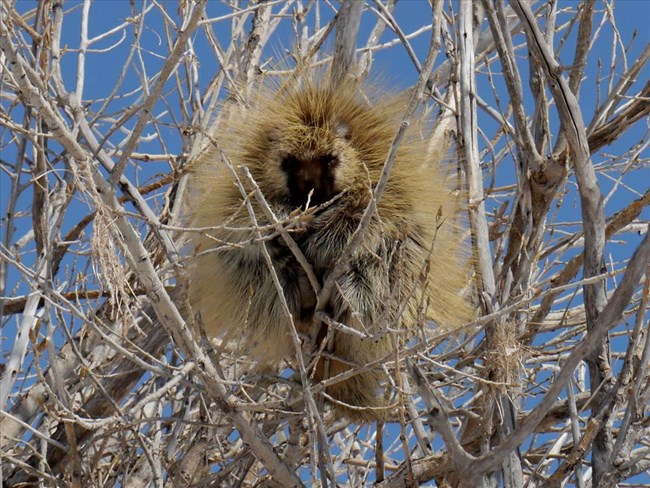The image features a porcupine perched atop a tangle of light beige and grayish tree branches, notably devoid of leaves, suggesting wintertime. The branches are wildly matted and appear dry and dead, creating a dense canopy that almost obscures the light blue sky behind them. The porcupine, with its spiky, sharp-looking fur, is huddled on a thin branch, holding onto another. Its face is darker around the muzzle and eyes, with a tan forehead and top of the head, while its chest displays a mix of black and white fur. The rest of its body is tan with a dark brown undercoat. The porcupine is looking directly at the camera; its expression is neutral, neither menacing nor friendly. Its positioning and the overall scene give an impression of a tranquil yet wild woodland moment.